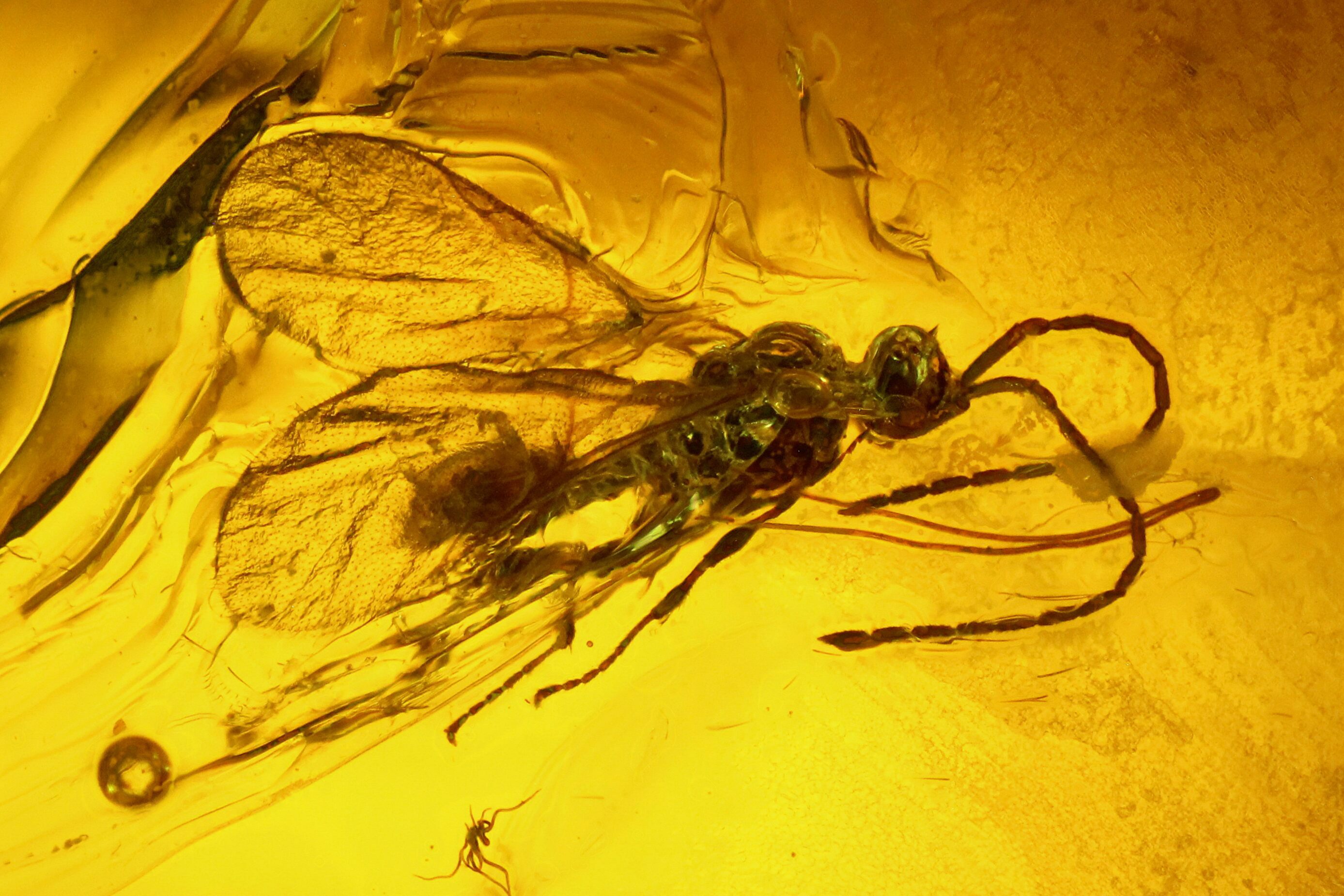The image presents a close-up view of an insect resembling a fly or possibly something in the wasp family, appearing to be encased in amber. The background is a bright, rippled yellow that is quite vibrant and uneven, especially notable on the left-hand side. Centered in this horizontal rectangular image is a large insect with a round head featuring two long, segmented brown antennae that curve underneath its head. Its body showcases various shades of green, dark brown, and black, with distinguishable clear wings that have brown edges, allowing the yellow background to be seen through them. The insect's legs are folded beneath its body, adding to the impression of being trapped. Below this larger insect, there is a much smaller creature, likely another insect, with identifiable thin arms and legs, further emphasizing the trapped-in-amber-like appearance of the scene.